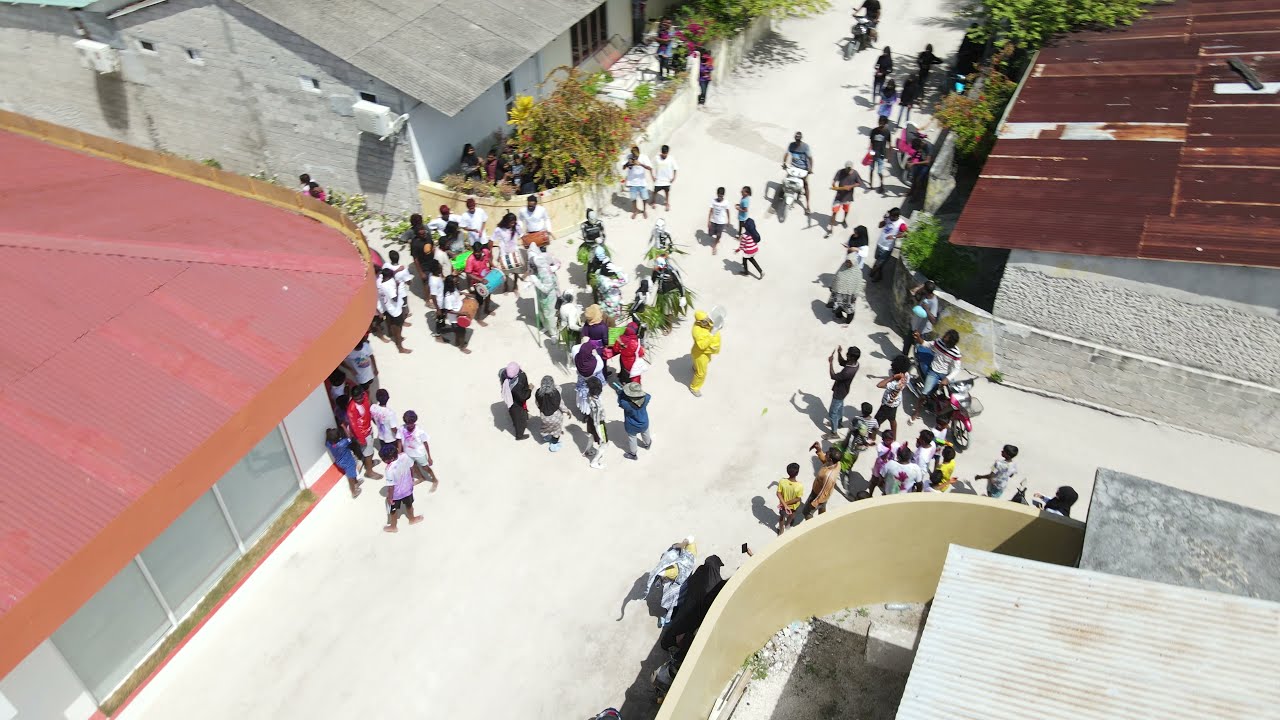An aerial photograph captures a bustling scene of schoolchildren, aged approximately 6 to 12 years, and a few adults, in what appears to be a school setting located in India. The central focus is an intersection of packed white dirt roads within the school compound, bordered by four buildings with distinct rooftops: one red, two gray metal, and one rusted brown metal. The children, dressed in colorful clothing including hues of yellow, red, green, and mainly white, congregate and interact, suggesting they're either between classes or being dismissed for the day. Among them stands a notable figure—a gentleman in a bright yellow suit and matching turban, holding a paper. The sun shines brightly, casting light on the gravel walkways and the vibrant scene below.